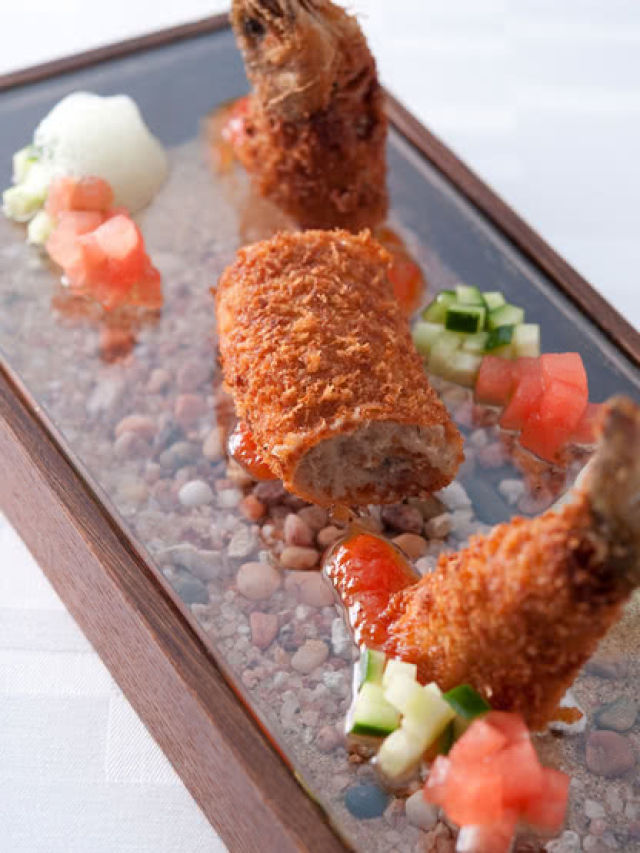The photograph captures a meticulously arranged food display, centralized on a glass platter with a wooden trim, resting atop a rectangular wooden basket filled with decorative, multi-colored rocks. The main attractions of the dish include pieces of what appear to be sushi or potentially fried chicken wraps. The reddish-brown exterior of the food is contrasted by the white interior, suggesting a blend of textures and flavors possibly featuring crab or lobster meat. Scattered around the central dish are finely diced vegetables, including green cucumbers, red tomatoes, and white onions. There is a hint of a red sauce drizzled on top, adding a vibrant splash of color. The overall presentation is enhanced by the sophisticated glass case and the sleek gray background, making the food the focal point of this image. This artistic culinary display exudes an air of elegance and creativity, making it a standout serving suggestion for any gourmet enthusiast.